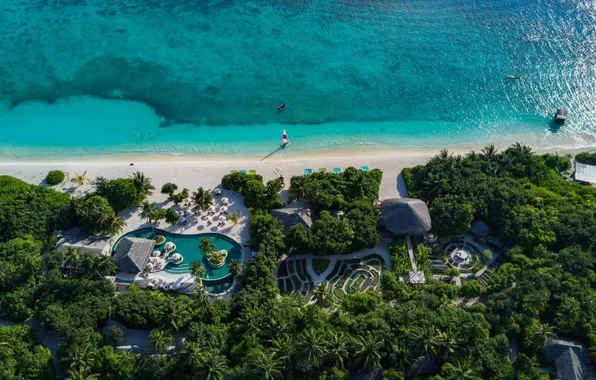This outdoor aerial color photograph showcases a picturesque beach resort surrounded by lush palm and tall green trees. The lower half of the image highlights the resort, featuring several homes, some with personal pools, and a complex garden area resembling a grass maze. Notably, the left side reveals a large pool with several protruding islands, while the right side features what appears to be a pavilion accompanied by a garden. The resort is canopied by an abundance of tree and greenery, suggesting an island locale. The central horizon line is marked by a sandy shoreline, beyond which lies the immaculate, teal-blue ocean, occupying the upper half of the image. The water, visibly clear to the ocean floor, is sparsely dotted by a singular, small sailboat situated near the center. Captured from a high altitude on a bright, sunny day, the photograph is devoid of visible people or text, evoking a serene and idyllic escape.